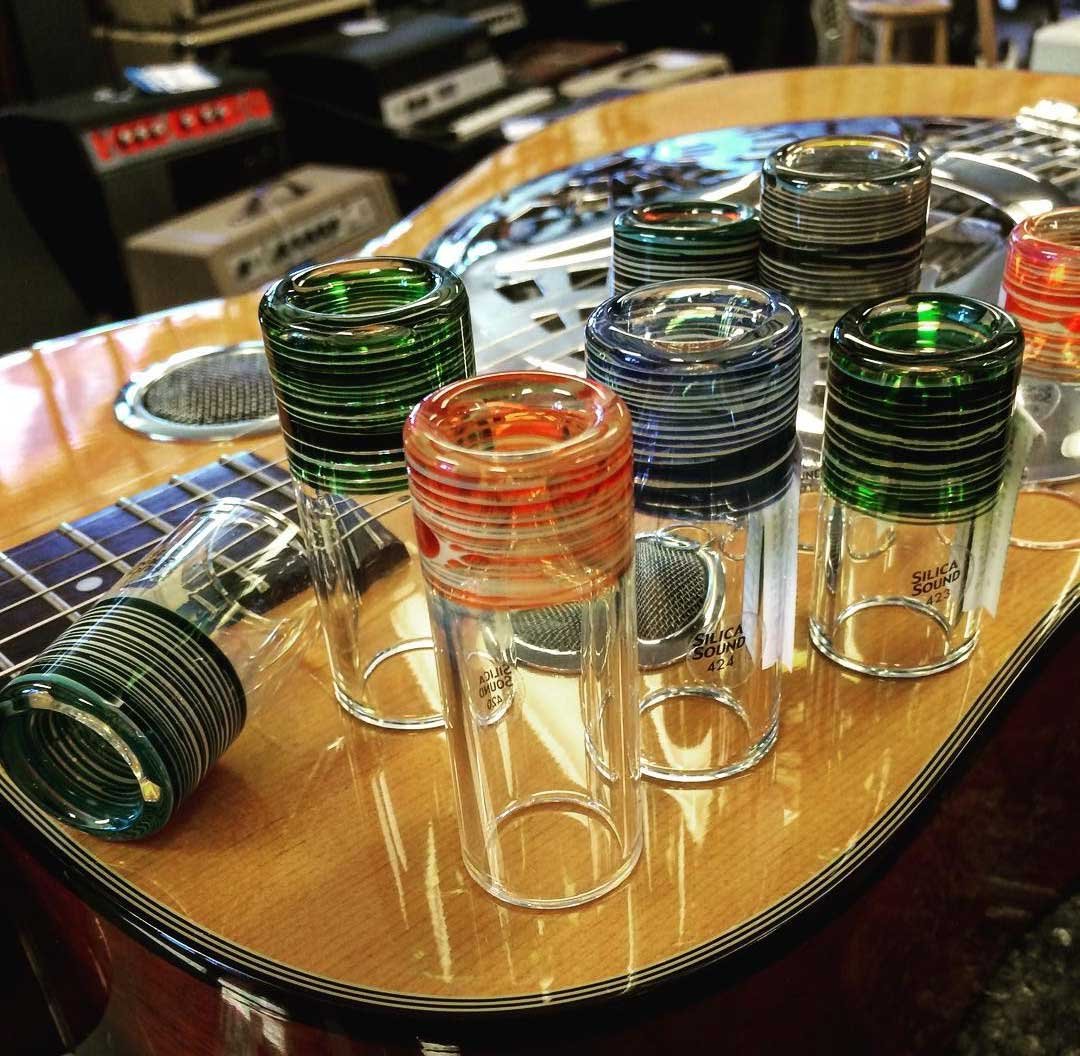The image depicts a polished, light brown, guitar-shaped table with a glass top, likely situated in a music shop. On this table, various clear drinking glasses, turned upside down, are adorned with the logo "Silica Sound" followed by different numbers like 423, 424, and 420. These glasses feature colored rims at their bottoms in hues such as green, black, blue, red, orange, and yellow, with some displaying swirly decorative designs. The glasses vary in size, height, and width. In the background, small amplifiers and other musical equipment are visible, hinting at a musical theme or a possible acoustic test setup.